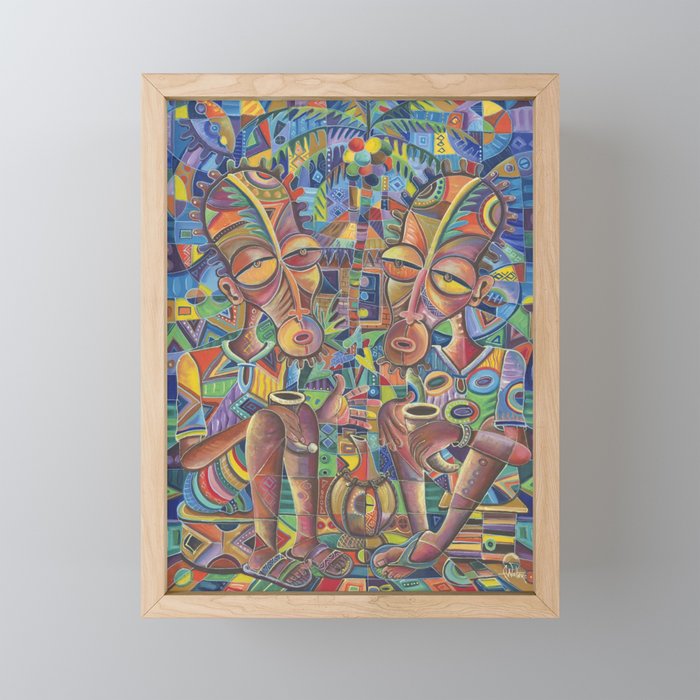The artwork, contained within a light tan wood frame around a smaller rectangle, is finely detailed and bursts with an array of vibrant colors. It depicts two seated figures with brightly colored, disproportionately large faces and eyes set against a mosaic-like background filled with small shapes of various hues. These figures, appearing to be African men with darker skin tones, wear shirts, shorts, and sandals. Each holds what resembles a horn or perhaps a drinking vessel in their hands. Between them on the ground lies an object that looks like a gourd or vase. The painting, though abstract, cohesively brings together a wealth of detail to form a vivid and dynamic piece without being overwhelming. The scene is set against a light gray wall, highlighting the rich complexity and cultural essence of the artwork.